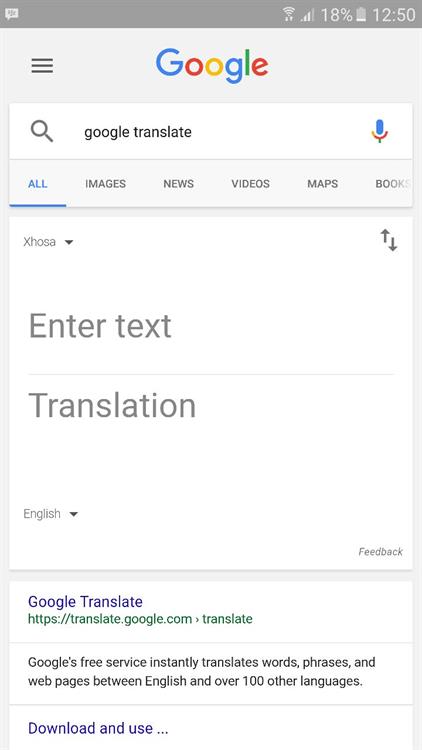This image depicts a tall, vertically-oriented screenshot of a mobile device interface, likely from an Android or iPhone. The top section includes a dark gray status bar with a speech bubble icon on the left, and standard status icons on the right: a Wi-Fi signal showing three out of four bars, an 18% battery life icon, and the current time displayed as 12:50.

Directly below the status bar, on a gray background, there are three black horizontal bars, recognized as a "menu" icon, positioned on the left. Next to it is the colorful Google logo, consisting of a blue capital 'G', followed by lowercase letters in red, yellow, blue, green, and red.

Centered just below the Google logo is a white search box featuring a gray magnifying glass on the left and the text "Google Translate" in black. To the right of the text box, there's a microphone icon. Beneath this search bar are navigation tabs in uppercase letters: "ALL" in blue with an underline, signifying the active tab, followed by "IMAGES", "NEWS", "VIDEOS", "MAPS", and "BOOKS" in gray, with the word "BOOKS" slightly faded out.

The main content area starts with a large white box. In the upper left corner, the word "XHOSA" is prominently displayed (capital 'X' followed by lowercase 'hosa'), denoting a language spoken in Southern Africa. Adjacent to it is a dark gray, downward-pointing triangle for selecting different languages. On the upper right, there are two dark gray arrows pointing up and down, possibly for swapping input and output languages.

In the center of the white box, large gray letters display the word "Inner text." Below this phrase, a faint gray line separates it from the word "translation." Another faint gray box below shows the word "English" with a downward-facing triangle for additional language options. In the lower-right corner of this white box, "Feedback" is written in gray letters.

Separated by a gray area, another long white bar appears with dark blue letters spelling "Google Translate." Underneath in green letters is the URL "https://translate.google.com" followed by a gray, sideways-facing triangle and the word "translate."

Further down, separated by a faint gray line, a brief description reads, "Google's free service instantly translates words, phrases, and webpages between English and over 100 other languages," in black letters. A faint gray line below this text segments from a final snippet featuring dark bluish letters with the words "download and use" followed by three dots, where the rest of the text is truncated due to the image cut-off.